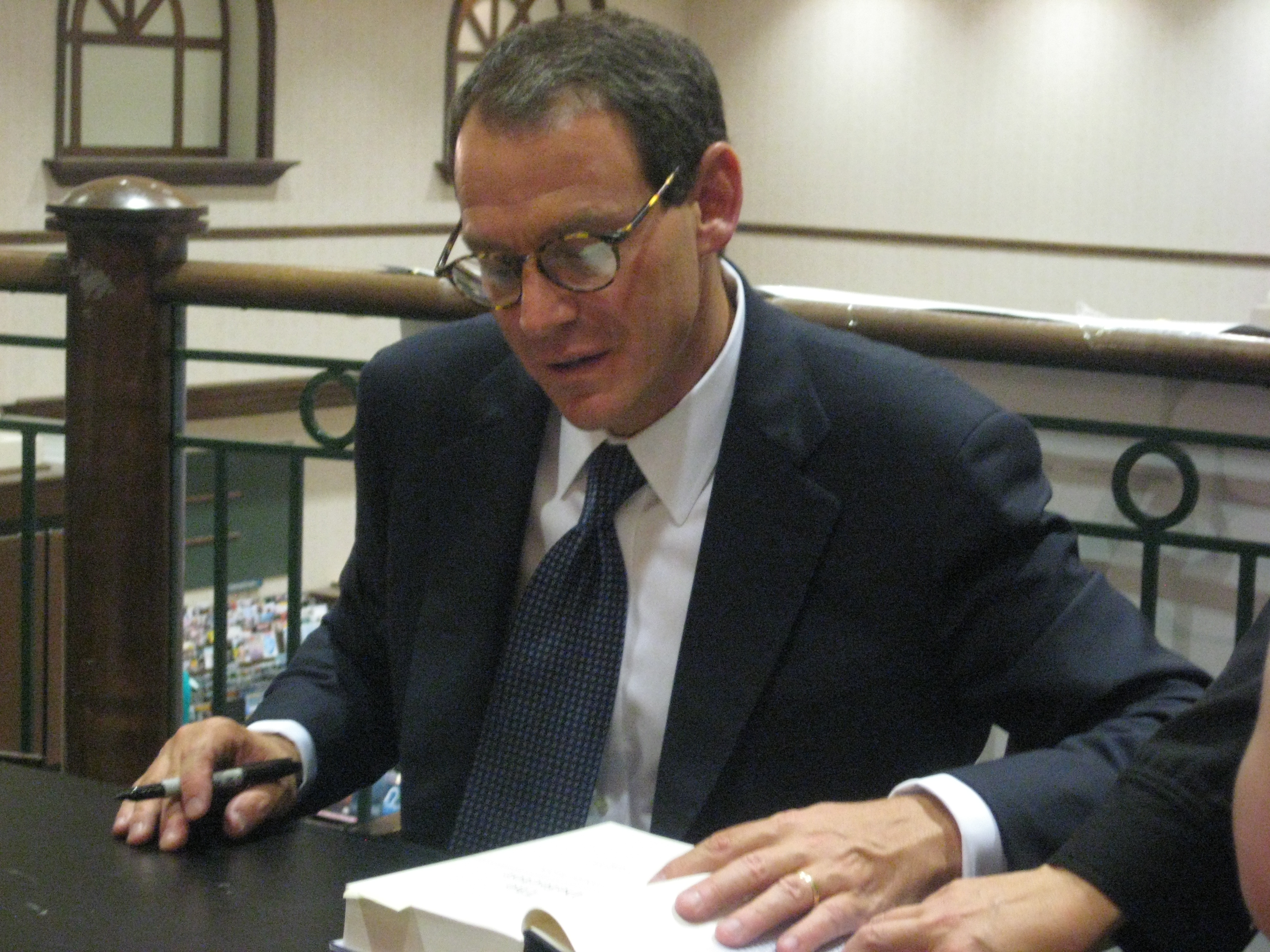This photograph depicts a middle-aged man, appearing to be in his 40s with short, slightly balding dark hair, wearing a dark blue suit paired with a white collared shirt and a dark blue and black checkered tie. He is sitting at a brown table, intently reading from a thick book with white pages. The man is holding a black and gray Sharpie in his right hand and wearing a wedding band on his left hand. He has glasses on and seems focused on the text in front of him. The setting looks like an older administrative building or library, characterized by white walls and brown window frames. In the background, there is a brown wooden railing with some metal elements, suggesting that the table is on a second-floor balcony overlooking what might be an office or library space below. Another person's presence is indicated by a hand with a black long sleeve, subtly visible next to the central figure. The overall atmosphere gives a professional or legal setting vibe.